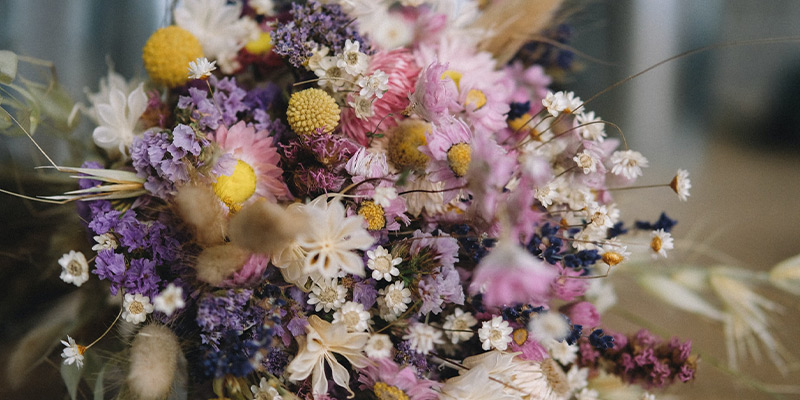A close-up photograph captures a vibrant bouquet of flowers, with the mid-ground in sharp focus. The composition features a harmonious mixture of colors: pink, purple, white, and touches of yellow. The bouquet includes small clusters of pink and purple flowers surrounding yellow centers, reminiscent of daisies, alongside larger white flowers with star-like appearances and yellow pom-pom centers. White wispy flowers and sprigs of lavender add a delicate touch to the arrangement. Some flowers and decorative stems appear dried, enhancing the bouquet's rustic, bohemian charm. The extreme foreground and background are notably out of focus, emphasizing the intricate details and colors of the floral assortment.